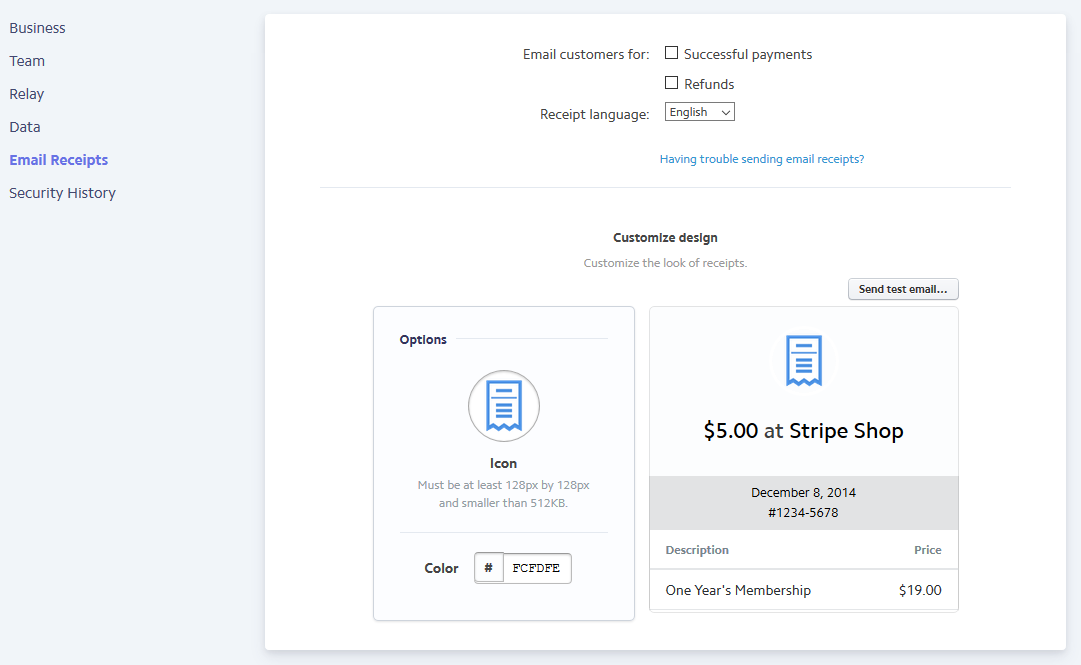This horizontal image resembles a screenshot from a user interface that can be viewed on a computer or digital device. The background features a blue-gray tone, with a white box occupying the right-hand side. In the upper left-hand corner, there are clickable options listed in black text: "Business," "Team," "Relay," "Data," "Email Receipts" (highlighted in blue, indicating it is the selected option), and "Security History."

Within the white box, there is a section titled "Email Customers For," followed by two unchecked boxes labeled "Successful Payments" and "Refunds." The "Receipt Language" is set to English, and beneath that, there's a clickable blue text reading "Having trouble sending email receipt?"

A horizontal dividing line separates this section from the next. Below the line, in bold black and gold text, it says "Customize Design." Additional options include "Customize the look of receipts" and a gray button labeled "Send Test Email" for user interaction.

The lower portion contains two segments. The left part, titled "Options," features a circular icon prompt and guidelines for uploading an image: "You must be at least 128 pixels by 128 pixels and smaller than 512 KB." Below that, there’s a color selection option. The right part displays a historical transaction: "$5 at Stripe Shop, December 8, 2014," with details like transaction number, description, and the price "One-year membership: $19."